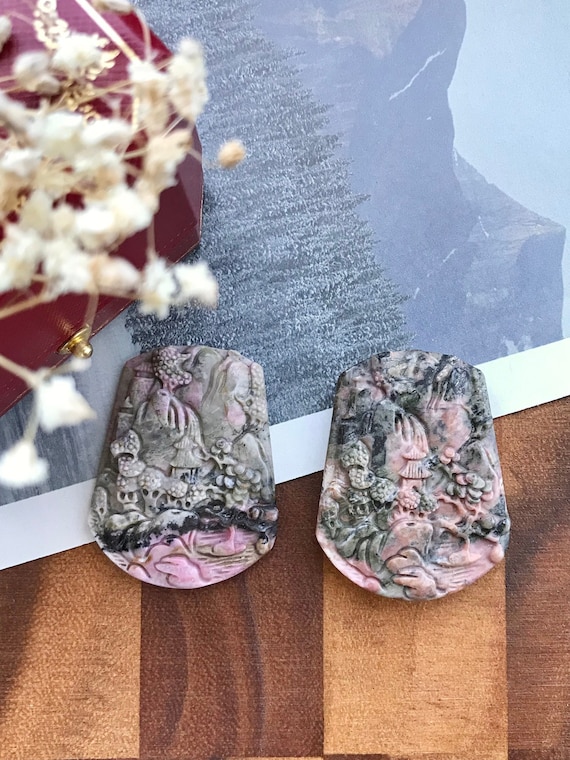This colored photograph captures a detailed top-down view of intricately carved stone pieces set on a wooden surface. The stones, appearing to be hand-carved and possibly for sale, feature a unique blend of white, gray, and pink hues, which is rare and striking. The carvings on these stones depict miniature scenes, likely of Asian origin, including designs of trees, buildings, and blossoms, with one stone displaying a distinctive oriental house. Positioned on the left side of the image is a red box adorned with white and gold floral patterns, resembling popcorn, under which lies a printed photograph of a mountainous landscape. This composition creates a visually rich tableau of mixed materials and textures, combining the smooth, variegated stones with the intricate, colorful box set against a light and dark brown wooden backdrop.